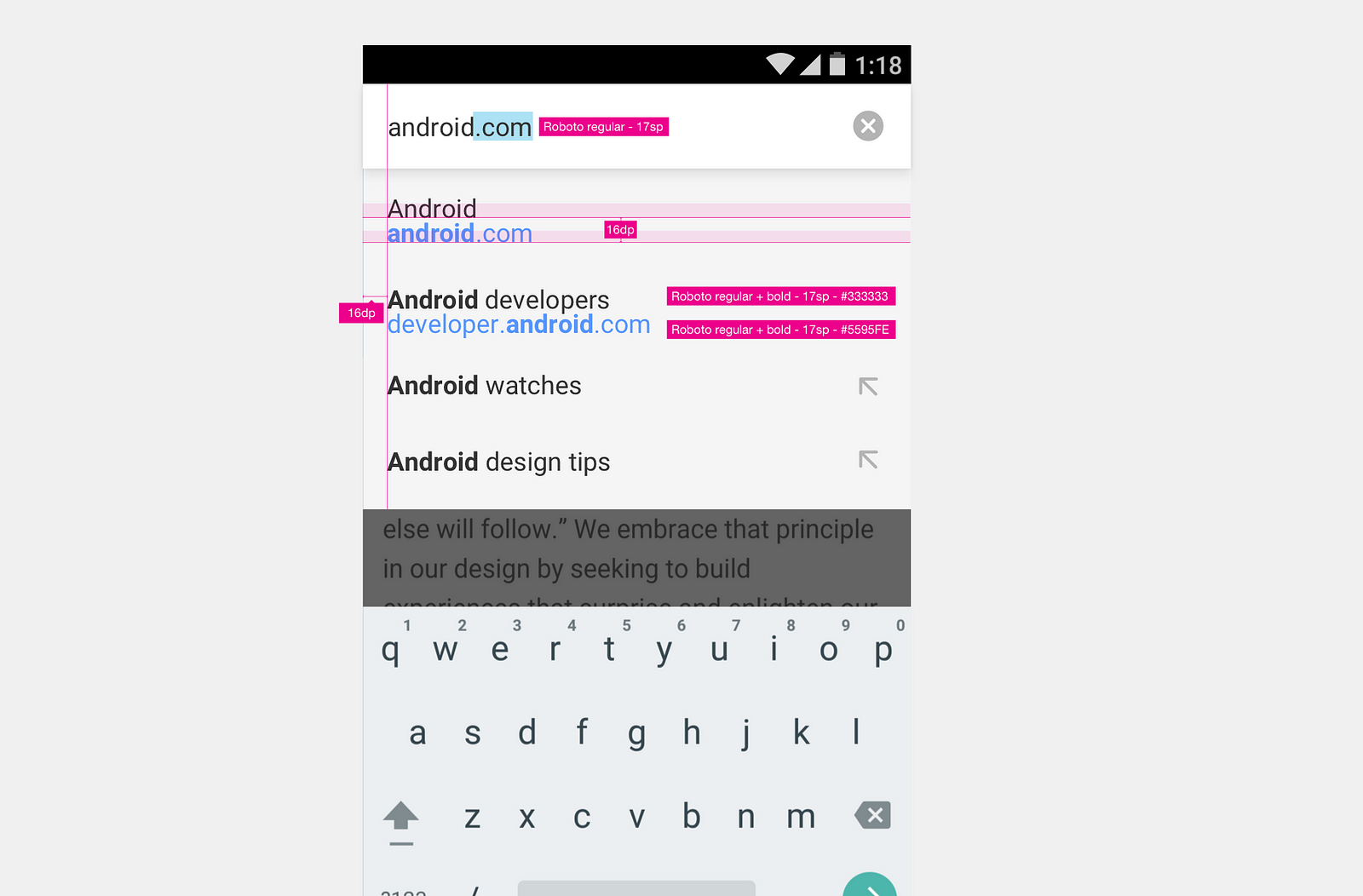The image depicts a smartphone screen displaying a webpage from android.com, highlighted in a teal color. The time at the top of the screen reads 1:18. Below the URL, enclosed in a pink box, there's an unreadable text element. 

Following this, in the middle section, there are various textual elements presented in an organized, aesthetic manner. The first line is the word "Android" rendered in bold black type, followed by "android.com" in blue type with a specification of 16 DP beneath it. Additional lines include "Android Developers" and to its right, "Roboto Regular and Bold - 17 SP," highlighting font specs. "Developer.android.com" is also displayed in blue, associated with the specification "Roboto Regular plus Bold - 17 SP". To the left of this, enclosed in pink boxes, are elements marked as 16 DP.

Further detailed segments include various design and font preferences. The visual hierarchy is accentuated by pink lines used as margins and borders dividing blocks of text. Specific words such as "Roboto Regular 17 SP" and "16 DP" are encapsulated within pink boxes.

Lower on the screen, the caption highlights the "Android watches" segment with navigation arrows pointing upwards and details like "Android design tips" also highlighted with arrows. A gray box below contains cut-off text, "else will follow. We embrace that principle in our design by seeking to build," hinting at partially visible content.

Intricately placed below the gray box is the phone's keyboard, indicating that the screenshot captures a moment of either editing or interaction on the website. The overall design and layout provide a structured and visually meticulous view into web design elements related to Android development.